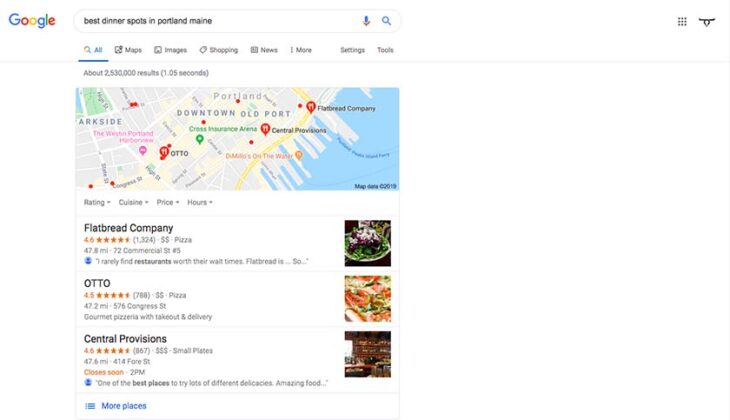This image is a detailed screenshot of the Google search page, capturing a query for "best dinner spots in Portland, Maine." At the top left corner, the Google logo is prominently displayed. It features the traditional Google lettering with a capital "G" in blue, a lowercase "o" in red, another lowercase "o" in yellow, an "l" in green, a red "e," and a final blue "g." Adjacent to the logo is the search bar with a microphone icon and a magnifying glass icon on the right side. The search query typed into the bar reads, "best dinner spots in Portland, Maine."

Below the search bar, there is a navigation menu offering various tab options such as "All," "Maps," "Images," "Shopping," "News," and "More." The "All" tab is currently selected. Further to the right, additional options are available for "Settings" and "Tools." Directly beneath these tabs, the page indicates there are approximately 2,530,000 search results retrieved in 1.05 seconds.

The image also includes a map of the Portland, Maine area, highlighting several restaurant locations with red pins featuring a fork and knife icon, representing dining spots. Below the map, there is a list of restaurant suggestions, starting with Flatbread Company, which has earned a rating of 4.6 stars from 1,324 reviews. The next on the list is Otto, with a 4.5-star rating from 788 reviews. Lastly, Central Provisions is featured with a 4.5-star rating from 867 reviews.